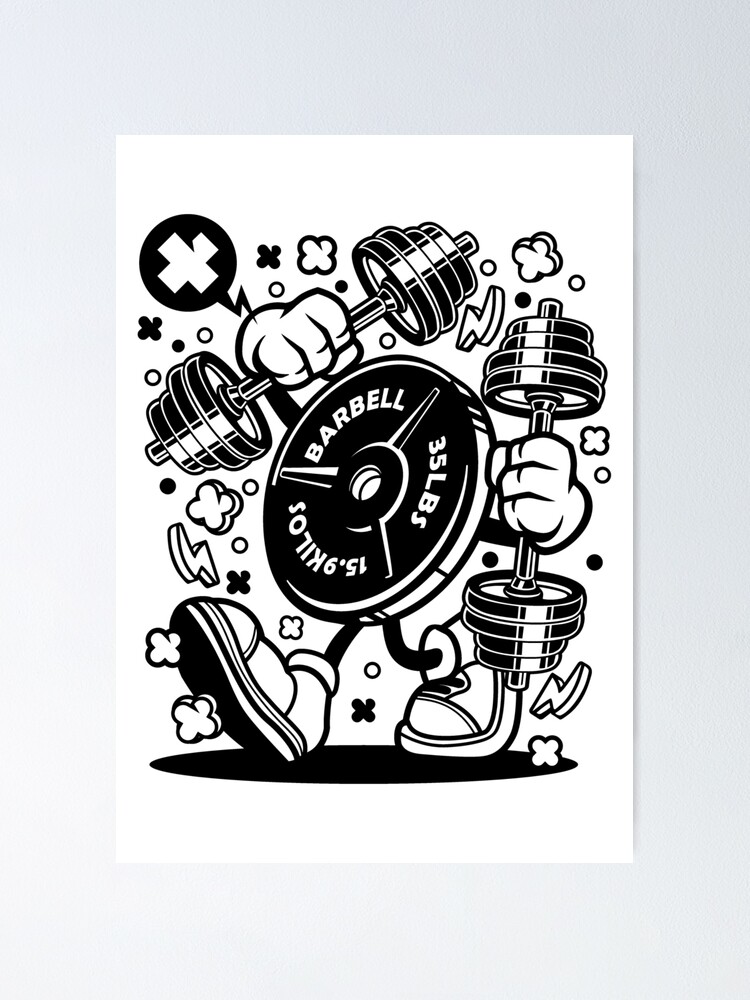This black-and-white illustration depicts a unique and whimsical scene. At the center is a round barbell with a hole in the middle, labeled "barbell, 35 pounds, 15.9 kilos." This anthropomorphic barbell has arms and legs, each foot clad in white shoes. In its hands, it lifts traditional dumbbells, one in each hand—an amusing pun on a weight lifting weights. As it walks, clouds of smoke and lightning bolts surround it, suggesting intense exertion or fatigue, further emphasized by a large X marker near its right hand. This image appears to be a poster, combining humor and the theme of fitness, highlighting the intensity and effort involved in working out.